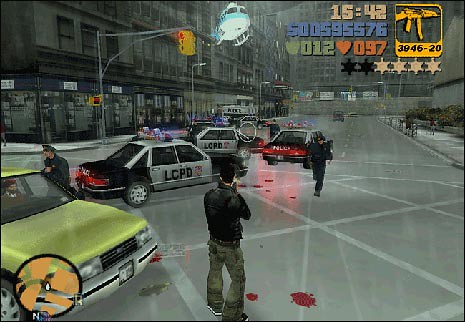This image is a detailed screenshot from an early Grand Theft Auto game, possibly Grand Theft Auto 3. It depicts the protagonist in a third-person shooter mode, sporting a black leather jacket and camo jeans. Positioned in the middle of a bustling intersection, the scene is set during what appears to be a rainy night. 

Adjacent to the character is a parked yellow taxi, and to the left, a partially visible light green car nose is seen. Directly facing him are several black-and-white LCPD police cruisers, with small in-game police officers pointing their guns at him. Red bloodstains can be spotted scattered on the gray street, heightening the sense of chaos. 

The protagonist is armed with a Tommy gun, facing away from the viewpoint, presumably firing towards the approaching police. Above them all looms a police helicopter near a traffic light. The in-game HUD displays crucial elements like the time, 15:42, and a round minimap at the bottom left corner. The character has accumulated four out of six police badges, indicating a high wanted level, and twelve hearts, possibly representing health.